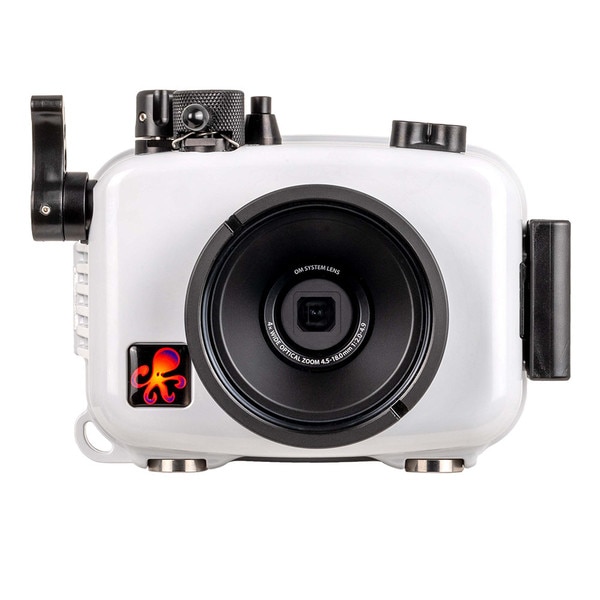In this detailed image, we see a close-up photograph of a white underwater camera set against a white background. The camera itself has a sturdy, robust design with a hard white shell, indicative of its waterproof capabilities. At the very center of the camera, there's a prominent black circular lens, which has "Olympus Lens" inscribed at the top. Below the lens, it reads "4X Wide Optical Zoom 4.5-118mm, 1:2.0-4.9".

The camera's rectangular shape is curved on all four sides, and it features several industrial-grade black knobs on top, a lever on one side, and a hinge on the other, ensuring it is sealed securely for underwater use. There's also a push button for taking photos. On the bottom left, a black label displays a fluorescent-colored octopus, adding a touch of character to the otherwise pristine white device. Additionally, there's a circular cut-out on the bottom right, likely intended for attaching a camera strap. The image illustratively captures the camera’s robust and functional design, suited for underwater photography.